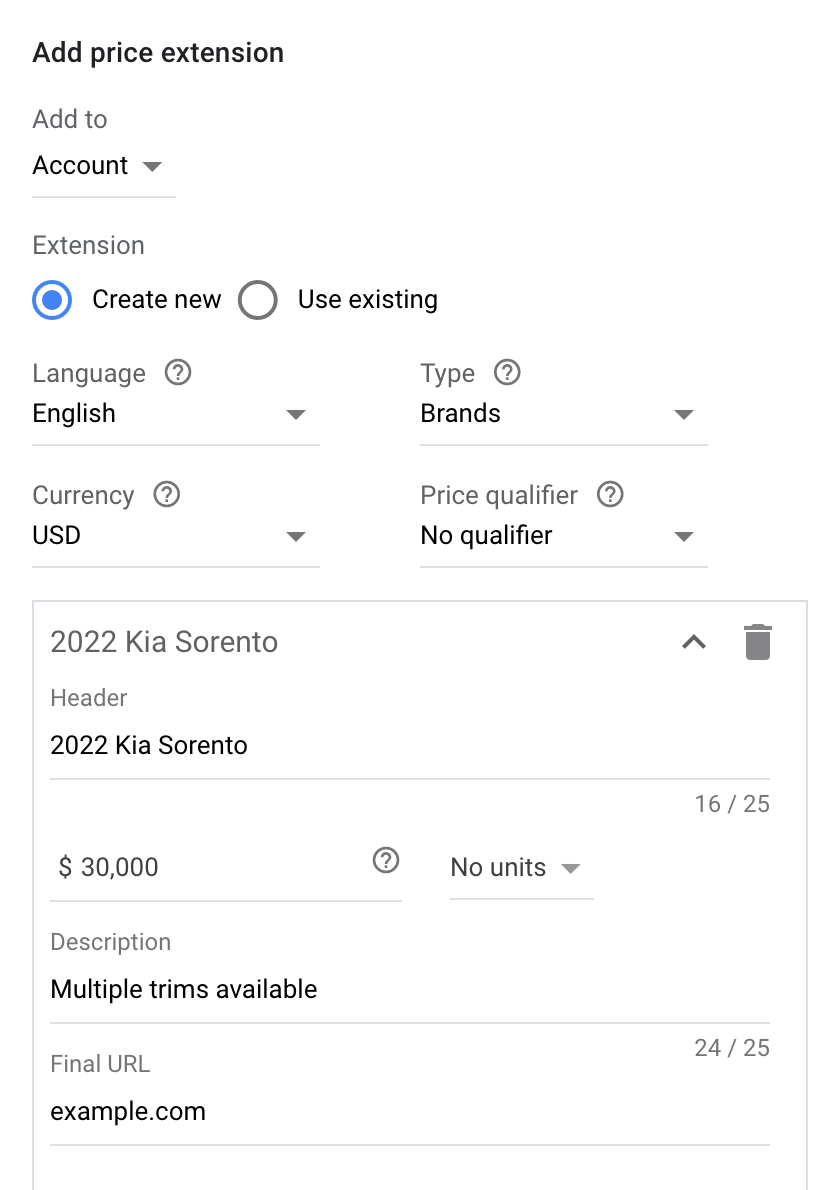The image displays a form against a white background titled "Add Price Extension." The form is structured as follows:

1. At the top, the section labeled "Add to" features a drop-down menu currently set to "Account."
   
2. Below, the "Extension" field allows selection between "Create new" or "Use existing," with the option "Create new" currently selected, indicated by a blue circle.

3. The "Language" field is set to "English."

4. Adjacent to this, the "Type" field is set to "Brands."

5. The "Currency" field is set to "USD."

6. The "Price Qualifier" section shows "No qualifier" selected.

7. Beneath these settings, the "Header" field is filled with "2022 Kia Sorento," utilizing 16 of the allowed 25 characters.

8. The "Price" field displays "$30,000," with no units specified.

9. The "Description" field contains the text "Multiple trims available."

10. At the bottom, the "Final URL" field lists "example.com."

Each input field is clearly defined, allowing the user to specify details for adding a new price extension effectively.